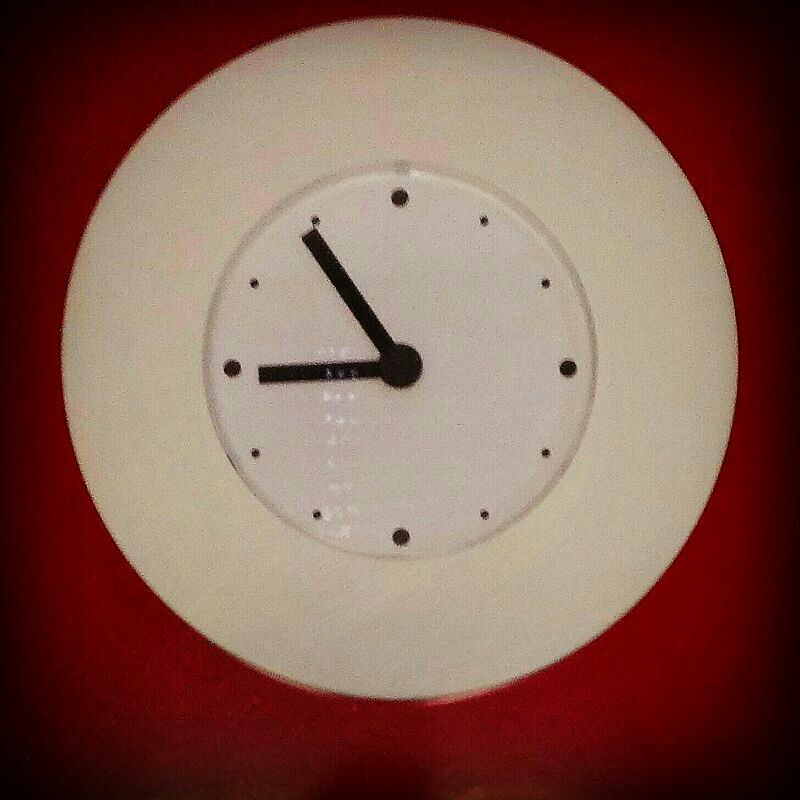A striking wall clock is displayed against a vibrant, ruby red backdrop, which has a subtle sheen suggesting it could be either wallpaper or a deep red painted surface. The clock features a thick, circular white frame that appears to be made of plastic. The clock face itself is pure white, devoid of traditional numbers. Instead, the hours are marked by minimalist black dots. Larger black circles denote the 12, 3, 6, and 9 positions, while smaller black dots represent the other hours. The clock's minute and hour hands are simple, thick black rectangles, with a slight sheen reflecting off their surfaces.